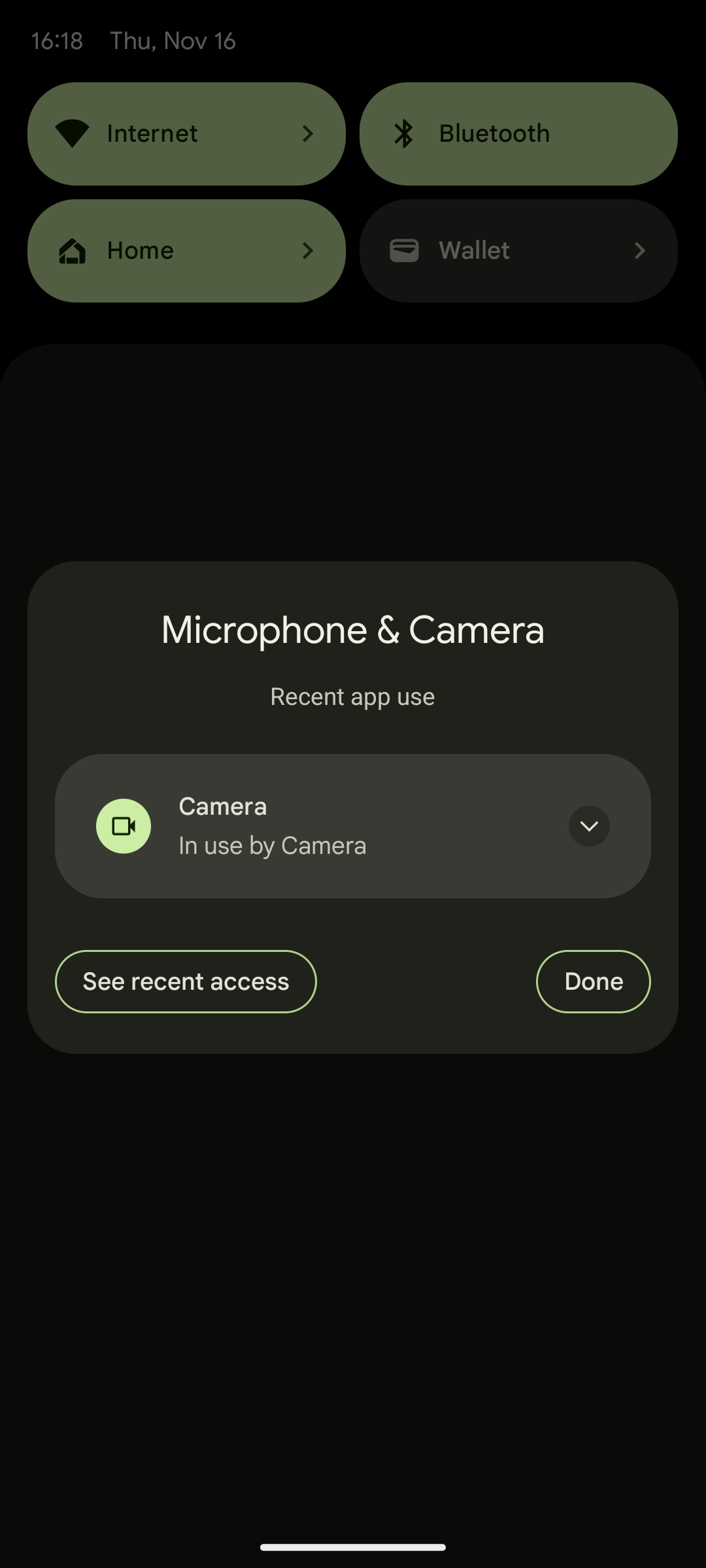The image is a phone screenshot taken at 16:18 on Thursday, November 16th, as indicated by the white-colored text at the top left. The top middle portion features four icons and their corresponding categories: "Internet" with a Wi-Fi signal icon, "Bluetooth" with a Bluetooth icon, "Home" with a house icon, and "Wallet" with a wallet icon. These categories are arranged in a 2x2 grid. The "Internet," "Home," and "Bluetooth" bubbles have a greenish background with black text, while the "Wallet" bubble features white text on a grayish-black background.

Centrally located in the image is a square notification bubble that reads "Microphone and Camera, recent app to use." Below this main text, a smaller boxed area identifies "Camera, in use by camera." At the bottom of this notification, there are two actionable options: "See recent access" on the left and "Done" on the right.